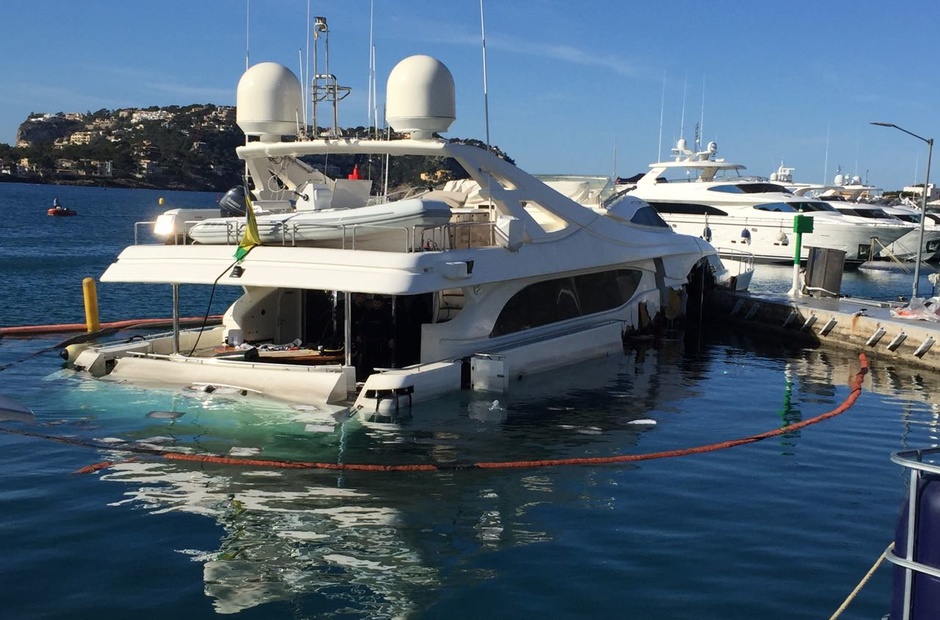In this detailed photograph, we see a vivid oceanic scene captured on a sunny day with a clear blue sky dotted with wispy clouds. Dominating the foreground is a white yacht, appearing luxurious yet half-submerged in the dark blue water, with a distinctive orange safety rope encircling it. This unfortunate vessel, moored at a dock visible at the right side of the frame, has its side window almost entirely below the water level, indicative of its critical condition. Surrounding this yacht are several other smaller, well-appointed white boats, suggesting a posh marina.

The harbor extends into the distance where an island with hilly terrain, crowded with buildings, creates a picturesque backdrop. Above the yacht, you can see a raft and a sophisticated twin radar system, signaling that this is an expensive, likely million-dollar vessel. On the left side of the image, near the distant shoreline, a red buoy adds a splash of color to the marine palette. The scene is devoid of any human presence, amplifying the yacht's silent distress and the serene, yet somewhat eerie, atmosphere of a quiet and sunny day in a bustling but tranquil harbor.